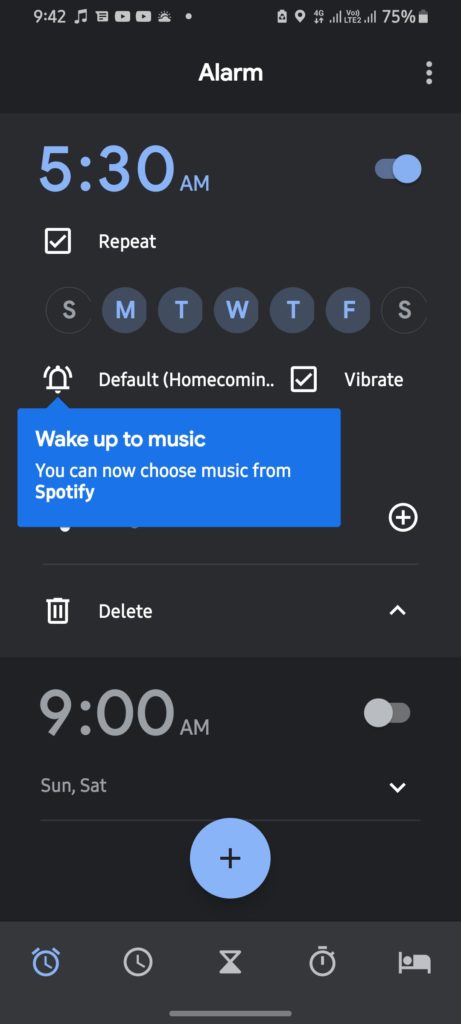The image depicts a smartphone screen displaying the alarm settings page. In the top left corner, the time is shown as 9:42 AM, accompanied by a "music mode" icon. To the right, there are paragraph and play button icons whose specific functions are unclear. The status bar along the top right shows various indicators: a phone battery icon, a pen icon, a 4G network indicator, Wi-Fi strength bars, and a battery percentage at 75%.

Below the status bar, the screen is divided into sections. The primary focus is on an alarm set for 5:30 AM. This section includes an "Enable" button, and indicates that the alarm is set to repeat on specific days, marked by the initials: S (Sunday), M (Monday), T (Tuesday), W (Wednesday), T (Thursday), F (Friday), and S (Saturday). There is a white check mark next to "Repeat" to show it's active.

Further down, there is an alarm bell icon next to a speech bubble with a blue background that reads, "Wake up to music - You can now choose music from Spotify." Below this, the word "Homecoming" is displayed, suggesting a song choice, followed by the "Vibrate" option for the alarm. 

At the bottom of this section, there are icons for deleting the alarm, represented by a trash can with an arrow, and a second alarm set for 9:00 AM. The 9:00 AM alarm section shows an "Enable/Disable" toggle, which is currently off, and indicates it is active on Sundays and Saturdays.

Finally, at the very bottom, there are additional icons for setting new alarms or timers: a big plus sign inside a circle, an alarm clock, a regular clock, an hourglass, an additional clock, and a bed icon.

The overall layout is clean and structured, providing all essential alarm setting options prominently for easy access.